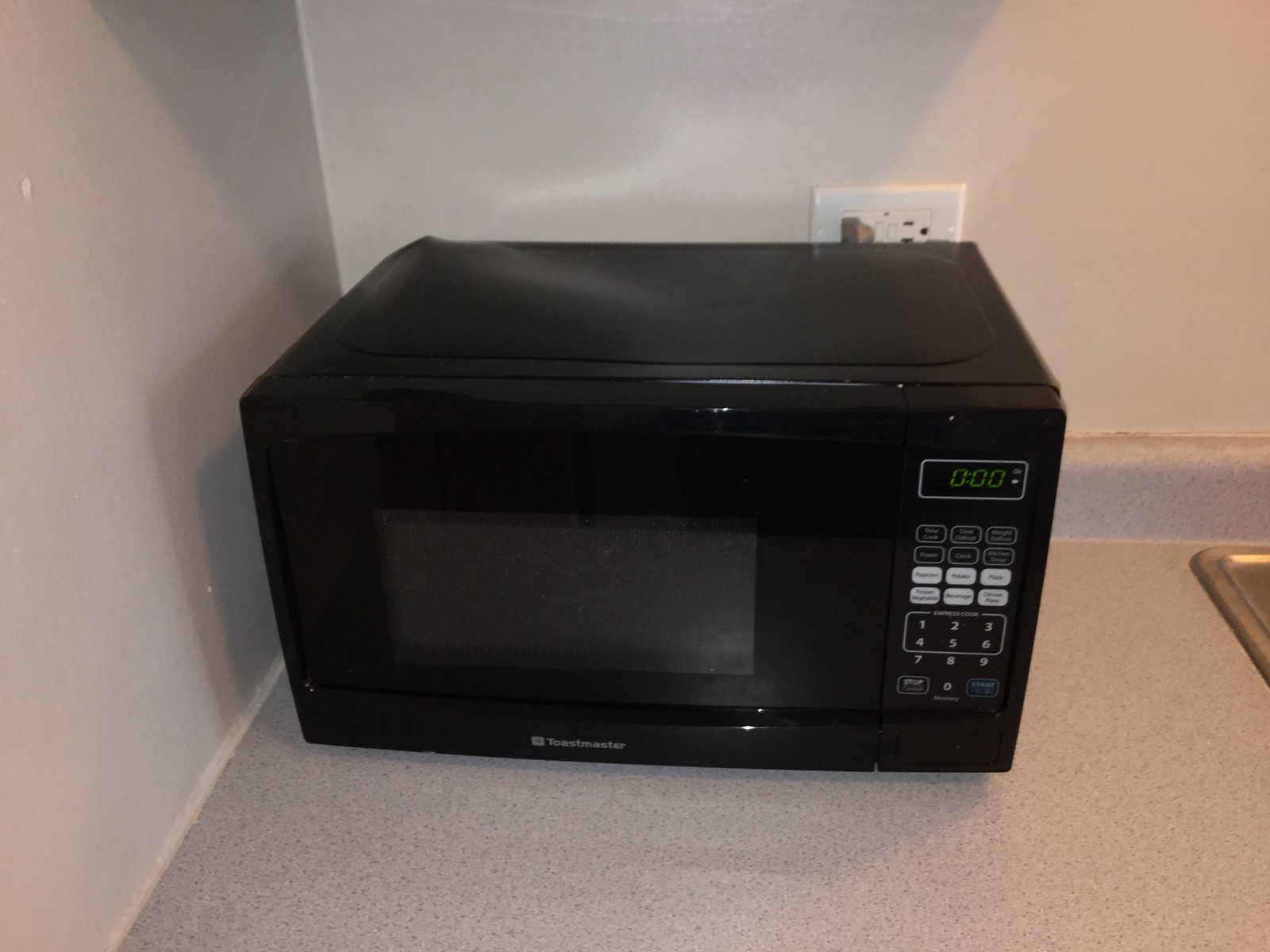This detailed photograph captures a black Toastmaster microwave situated in the corner of a kitchen countertop. The microwave features a clear glass window on its front door, through which the interior is visible, though it is currently turned off. The door also displays the brand name "Toastmaster" in white text at the bottom center. To the right of the window, there is a control panel with an array of white buttons and a green LED display that shows "0:00." 

The microwave is placed on a speckled gray countertop, beneath which parts of a stainless steel sink are visible at the right edge of the image. This countertop extends to form a corner, bordered by two walls meeting at a 90-degree angle. The wall to the left appears grayish, while the one directly behind the microwave is an off-white or tan color. Behind the microwave, a white, sideways-oriented electrical outlet with a dark gray or brown plug inserted into it can be seen. The overall photograph focuses mainly on the microwave, providing a slightly overhead view of the appliance and surrounding area.